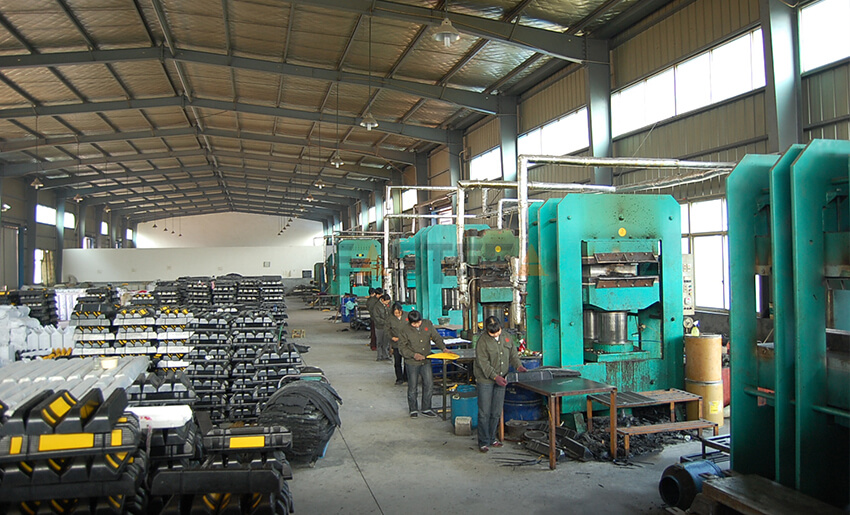The photograph captures the interior of a large manufacturing warehouse with a slightly sloping foundation-lined ceiling reminiscent of an airplane hangar. The scene is dominated by shades of gray and brown with splashes of teal green from the tall machinery lined up on the right side. These teal green machines, which feature a feeder with a metal mouth and a central compression chamber, are clumped together in groups of three and extend along the wall near the windows.

Assembly line workers, clad in gray jackets and jeans, some of whom appear to be Asian, diligently operate these machines. Six individuals can be seen in the photo, working at tables and handling the machinery as they produce unspecified items. The factory floor appears somewhat messy, with various items scattered beneath the machines.

On the left side, large stacks of black and yellow pallets and crates are neatly organized, ready for packing and shipping the products. These stacks are arranged in one direction rather than crisscrossed. Further back in the building, a white dividing wall is visible, and the entire space is illuminated by white hanging lights from the ceiling.